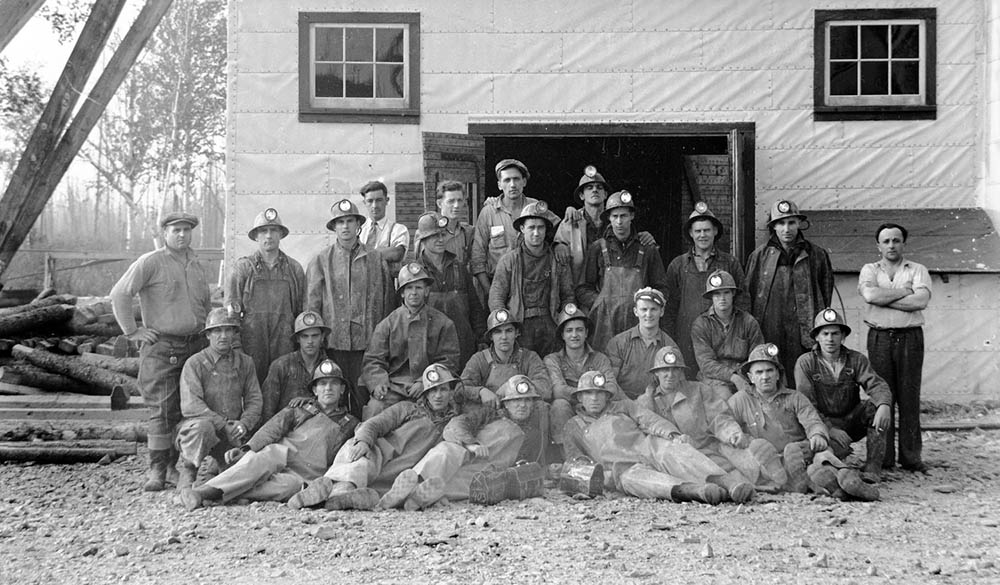The black-and-white photograph features a group of men, seemingly comprising both firefighters and miners, posing in front of an old-fashioned, white building. The building appears to have a material covering that ripples in the wind, suggesting it's not constructed from brick or cinder block. It has two six-pane windows with black shutters and a set of double doors that are wide open. 

The men are arranged in four rows: the first row is laying across the dirt ground, propped up on their elbows; the second row is kneeling or crouched; and the remaining two rows are standing. The ground beneath them is a rocky, dirt area, devoid of grass. To the left side of the image, cut logs are visible, along with some deciduous trees in the background. 

The men wear a mix of attire—some in overalls, hard hats with lamps, and various work uniforms, while others are dressed more casually, with one man in dress slacks and a white short sleeve shirt. There are men without hard hats, either bareheaded or wearing caps, and one man stands out at the far right in a tie and suspenders, without a uniform. At the far left, another man wears boots, rolled-up jeans, a long-sleeve shirt, and a felt cap. The photo captures a diverse group of working men, possibly from different professions, united in a single moment.